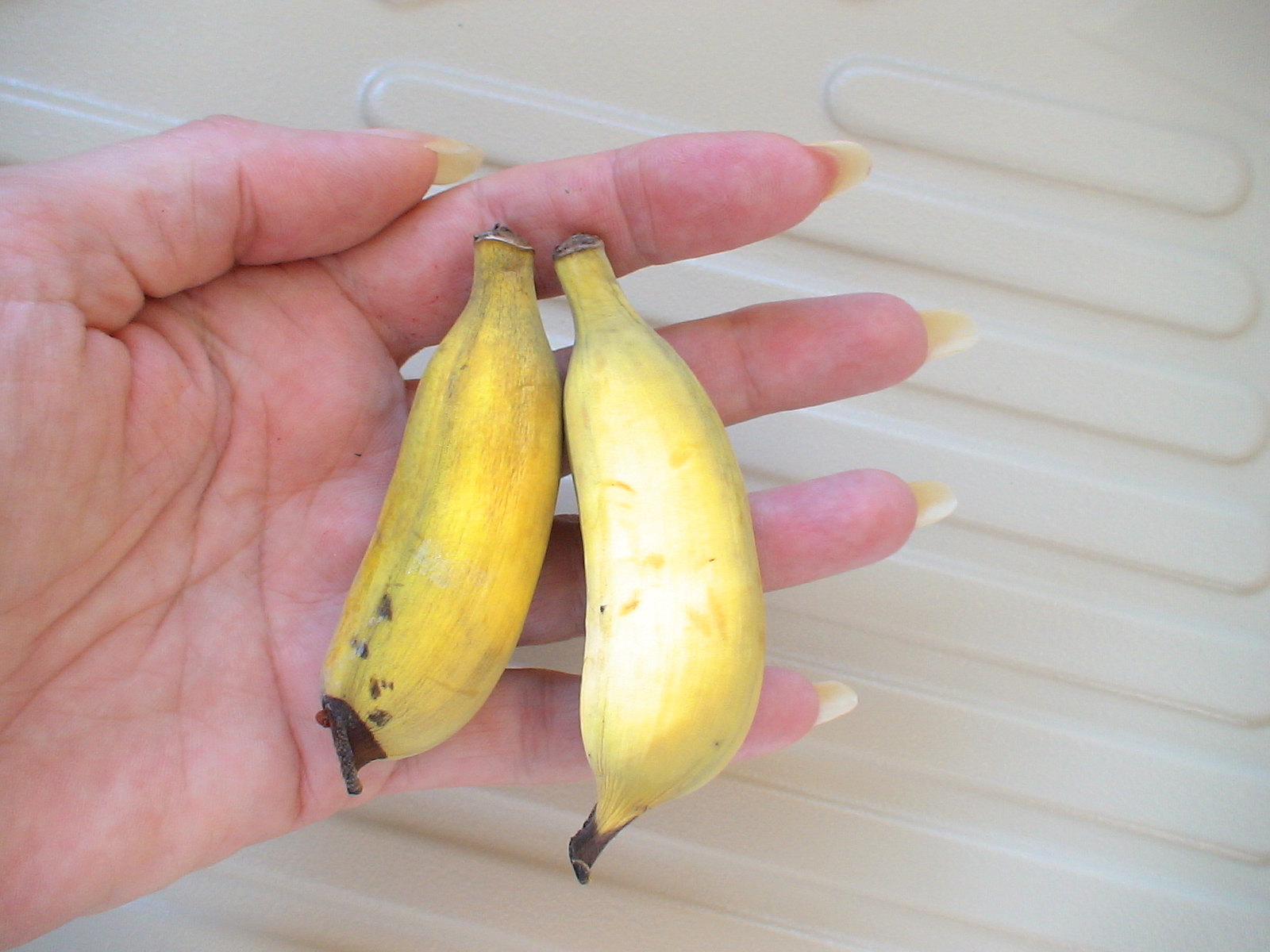In this detailed image, we see two very small bananas held in a person's hand, prominently displayed with a zoomed-in focus. On the left-hand side of the image, we observe the underside of the hand turned sideways, offering a horizontal point of view. The hand is white with a pinkish hue and features noticeable wrinkles on its underside. All five fingers and the thumb are clearly visible, with the nails showcasing a whitish-yellow underside.

The two small bananas are held within this hand. The banana on the left is slightly darker than the one on the right, which is highlighted by white light reflecting off its top. Both bananas have black-tipped ends, with the left one displaying a couple of black spots and a streak running through it. 

The background of the image is predominantly white, adorned with long, horizontal, oval-shaped elements that extend from the bottom, up the right-hand side, and across the top.